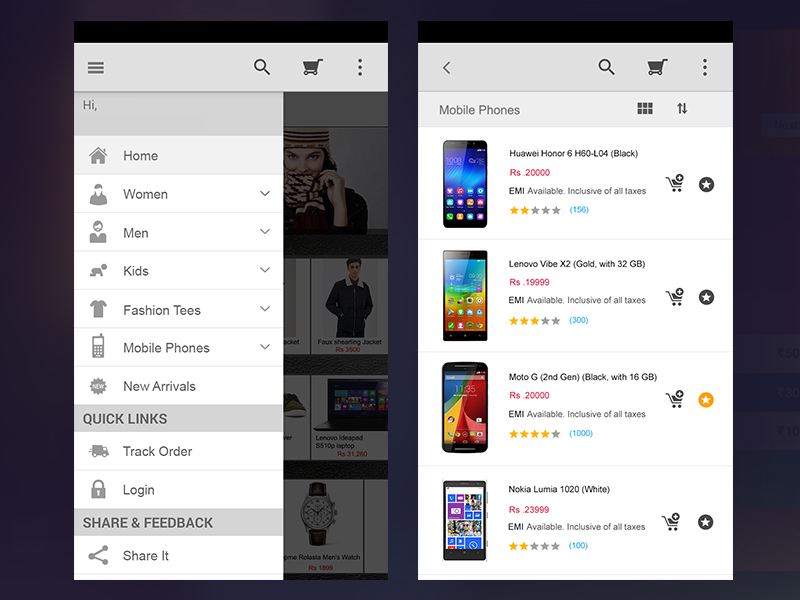This image features what appears to be two pop-up windows, initially giving the impression of mobile phone screenshots. The pop-up windows have a white background, with grey-topped headers positioned on the left side, adjacent to a kind of grey sidebar. The overall background of the image is almost black or very dark blue/grey, featuring darker edges at the top.

In the left window, there's an interface that includes a hamburger menu icon in the top-left corner, followed by a search icon, a cart icon, and three-dot menu. Below these icons, there's a pull-down list that includes the text "Hi" and is accompanied by grey icons next to grey text. The listed items are: Home, Women, Men, Kids, Fashion Tees, Mobile Phones, New Arrivals, Quick Links, Track Order, Log In, Share and Feedback, and Share It.

Underneath this, on the lower-right, there are images depicting a woman wearing a hat, a man in a jacket, a laptop, and a watch.

The right window shows a similar grey-topped bar. Below this bar, it is labeled "Mobile Phones", and it showcases four different mobile phones on the left panel:
1. Huawei Honor RX 2000: Two stars out of five, based on 15 reviews.
2. Lenovo Uber C3: Three stars, priced at 1999 in an unspecified currency.
3. Mito G Grey: Four stars with 100 reviews, priced at 2000 in the unidentified currency.
4. Nokia Lumia 120 White: Two stars out of five from 115 reviews, priced at 2299 in the same unidentified currency.